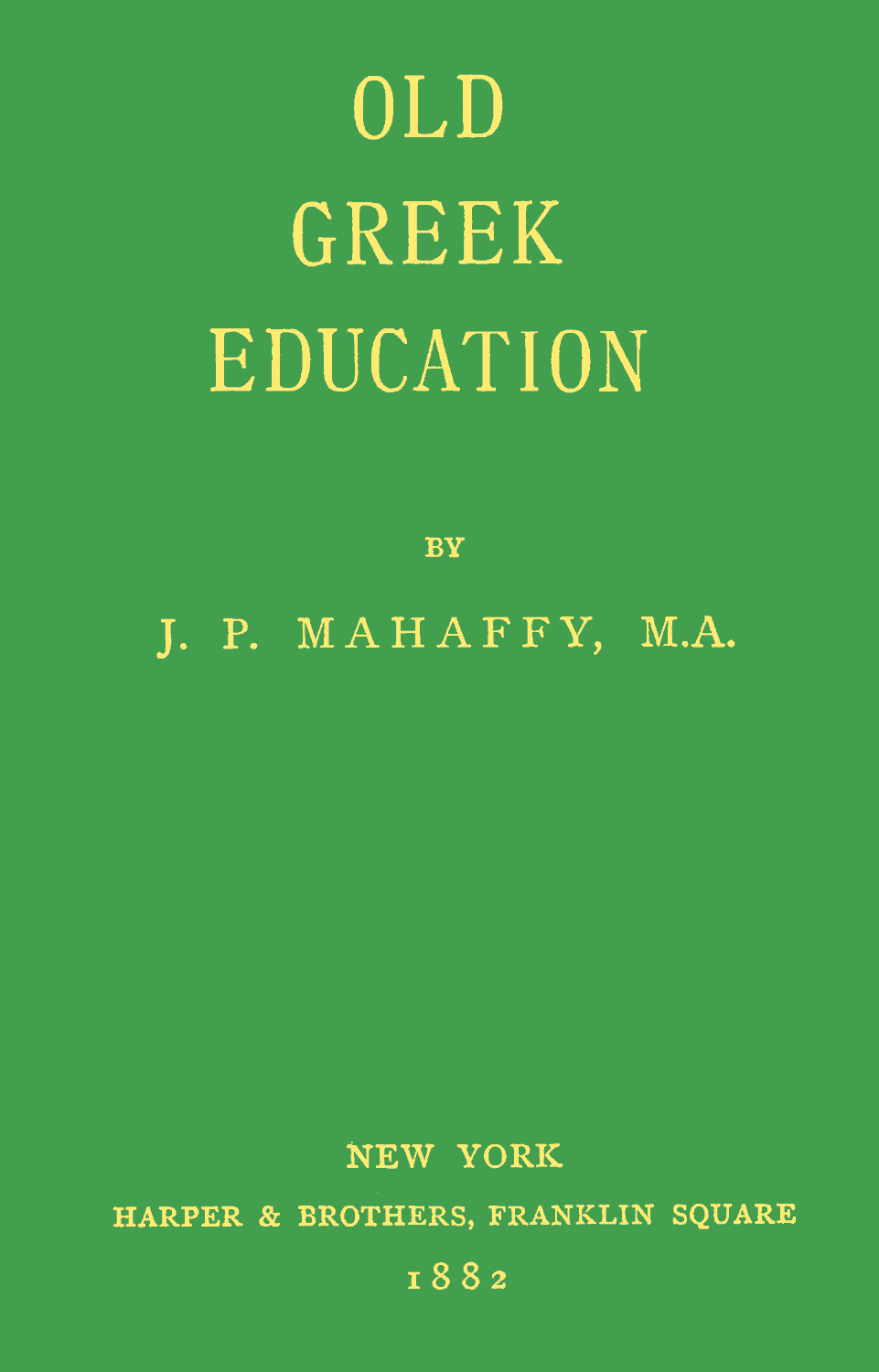The image depicts the cover of an old educational book titled "Old Greek Education" by J.P. Mahaffy, M.A. The cover is distinctly green with prominently embossed gold-yellow lettering. The title "OLD GREEK EDUCATION" is positioned centrally and is written in large, bold capital letters. Below the title, in slightly smaller but still bold capital letters, is the author's name, "J.P. MAHAFFY, M.A." Further down and also in capital letters, it reads, "NEW YORK," followed by "HARPER AND BROTHERS," and then "FRANKLIN SQUARE." At the very bottom of the cover, the publication year "1882" is inscribed. The overall design is minimalistic with no additional illustrations or decorative elements, focusing solely on the textual information.